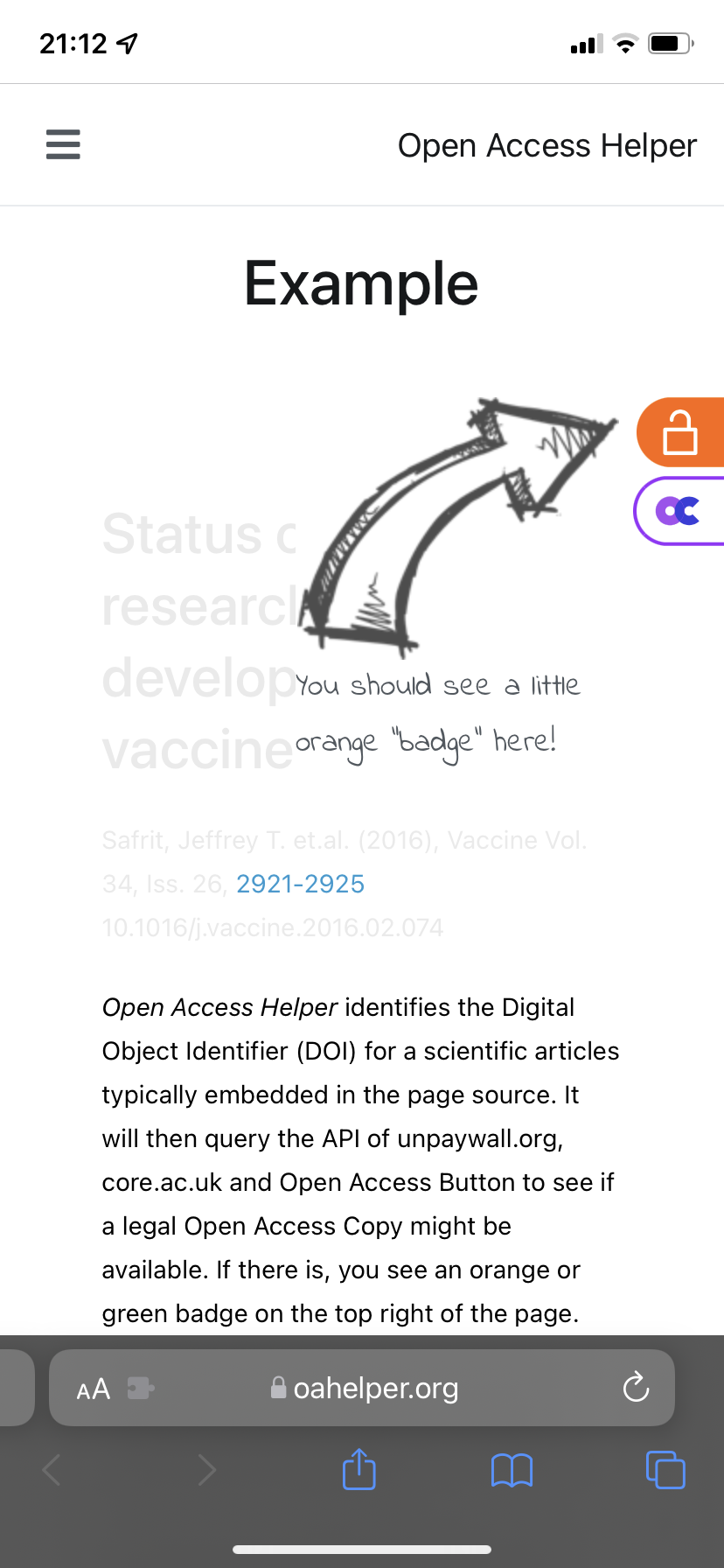The image is a screenshot taken on a mobile device, evidenced by the vertical orientation and various UI elements typical of a smartphone. The background is predominantly white. In the top left corner, the time is displayed as 21:12, and the battery indicator shows a charge of approximately 75%, not currently plugged in for charging.

On the right side of the screen is the text "Open Access Helper," and on the left side is a three-line icon representing a dropdown menu. Below these elements, the word "Example" appears in black text. An illustration of an arrow points to the right, indicating an orange badge. This badge features a small white lock icon.

Further down, there is a white tab with a purple border and the letters "O" (in purple) and "C" (in blue) conjoined. Underneath the main arrow, there's a gray heading that reads “Status: Research develop vaccine,” followed by some citations.

Beneath this heading, black text describes how the "Open Access Helper" identifies a Digital Object Identifier (DOI) for scientific articles, typically embedded in the page source. It further explains that the tool queries APIs from unpaywall.org, core.ac.uk, and the Open Access Button to check for the availability of a legal open access copy.